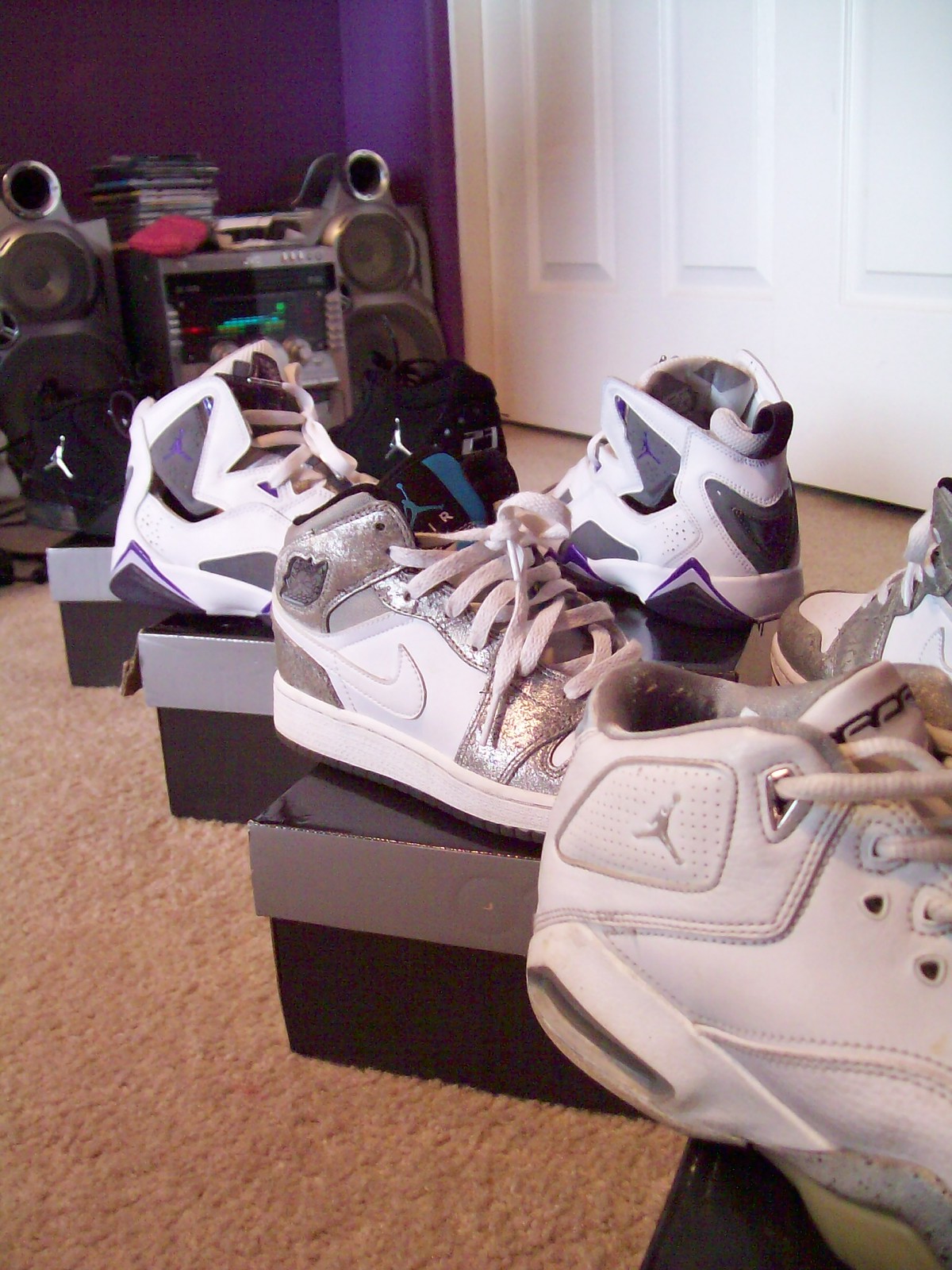This image features a close-up of three pairs of Nike shoes, neatly displayed on top of their original black and silver shoe boxes. The arrangement of the shoes forms two diagonal rows, creating a layered effect. The shoes closer to the camera include a mostly white pair with silver accents and white laces, a pair of all-white Air Jordans with a silver Air Jordan logo and white laces, and further back, a pair of Air Jordans with a combination of white, black, and purple hues. Additionally, in the second diagonal row, there is a pair of black Air Jordans with blue detailing. These shoes, appearing new and pristine, rest on a soft, light brown carpet. The room features purple walls and a visible lower part of a white door. In the background, a stereo system with a stack of CDs on top is flanked by two speakers, adding to the room's character.